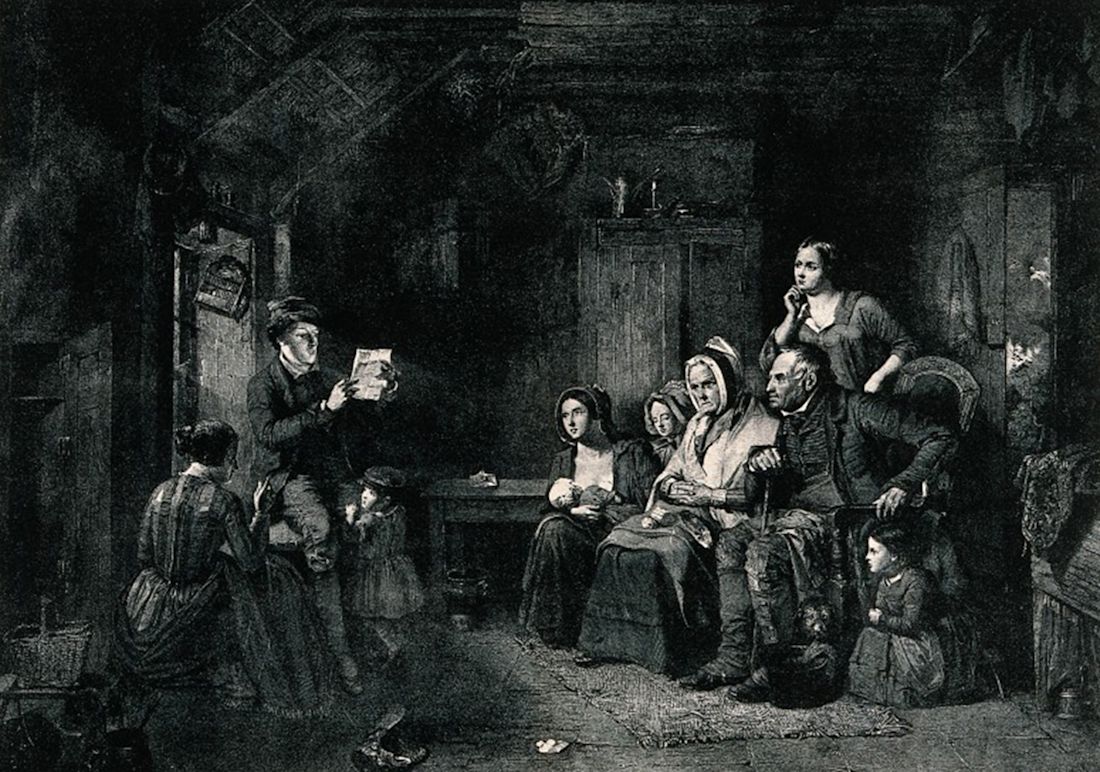In this horizontally aligned, large rectangular black and white image—likely an etching or detailed drawing—we see a family scene set in a worn stone structure, possibly from the 19th century. The setting resembles a living room with a door to the left and a cabinet or wardrobe behind the main subjects. The image shows a man on the left, standing and reading a document, likely illuminated by a nearby window. At his knee, a young child is positioned, while to his right, a woman is seated. She wears a long dress, and looks intently towards the man reading.

On the opposite side, on the right, are five or six family members, most of whom are seated. A man is leaning forward in an easy chair, holding a cane, with a woman beside him in a bonnet and long dress. A younger woman and a girl, both also in bonnets, sit nearby. Behind this group stands another young woman, all directing their attention to the man with the document. The ground appears to be covered with a rug or possibly hay, adding to the rustic feel of the scene. The expression on the gathered family members ranges from serious to stern, especially notable in the woman with the white hood, who displays an angry demeanor. The entire scene is rendered in contrasting black and white tones, enhancing the somber and timeless atmosphere of this historical moment.